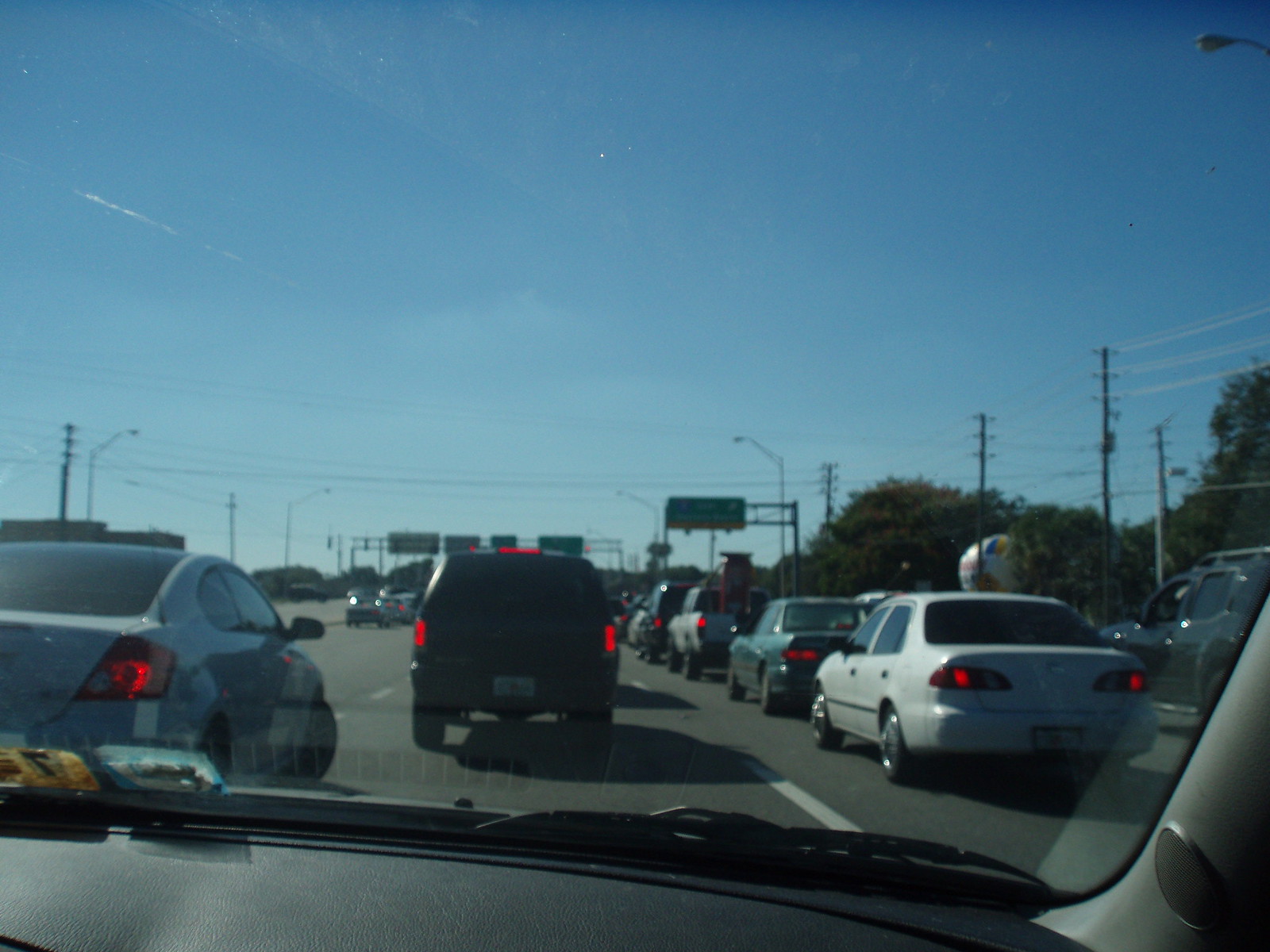This image depicts a congested three-lane highway under a clear blue sky, viewed from the front windshield of a car. Both sides of the highway are lined with overhead streetlights and telephone poles, which extend into the horizon. On the left side of the image, about a third of the way up, a hot air balloon floats above some bushes and trees. The traffic comprises various vehicles, including a gray car merging, a black SUV with tinted windows, and a light gray car on the left. Also, visible on the left is a blue car followed by a truck ahead. The brake lights of the cars in front are illuminated, indicating a stop-and-go situation. In the far distance, street signs for upcoming exits are visible. The far-right side of the image shows cars traveling in the opposite direction.